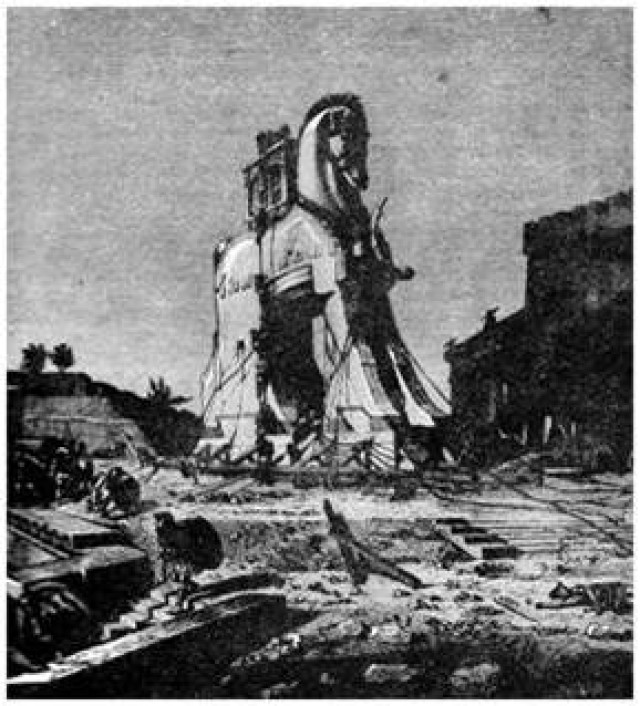This grainy black and white image depicts a monumental Trojan horse standing at the center of a construction site with a light-colored ground. The Trojan horse, about 60 feet tall, is prominently illustrated with its head facing slightly to the front and downward. It features a bristly mane on top and a wooden container with an arch on its back. The horse's front hooves slope down to a wooden platform supported by angled wood supports. Surrounding the horse, blurry outlines of a couple of people can be seen, resembling warriors with shields and helmets. To the right, there is a tall silhouetted building with crenellations halfway up, while the left side of the image showcases three distant palm trees and a hill with more trees. In front of the Trojan horse, steps lead down from the ground level, which is scattered with rocks and pebbles. The scene is detailed with additional elements such as ropes securing the structure and various blocks of wood placed in the bottom left corner.